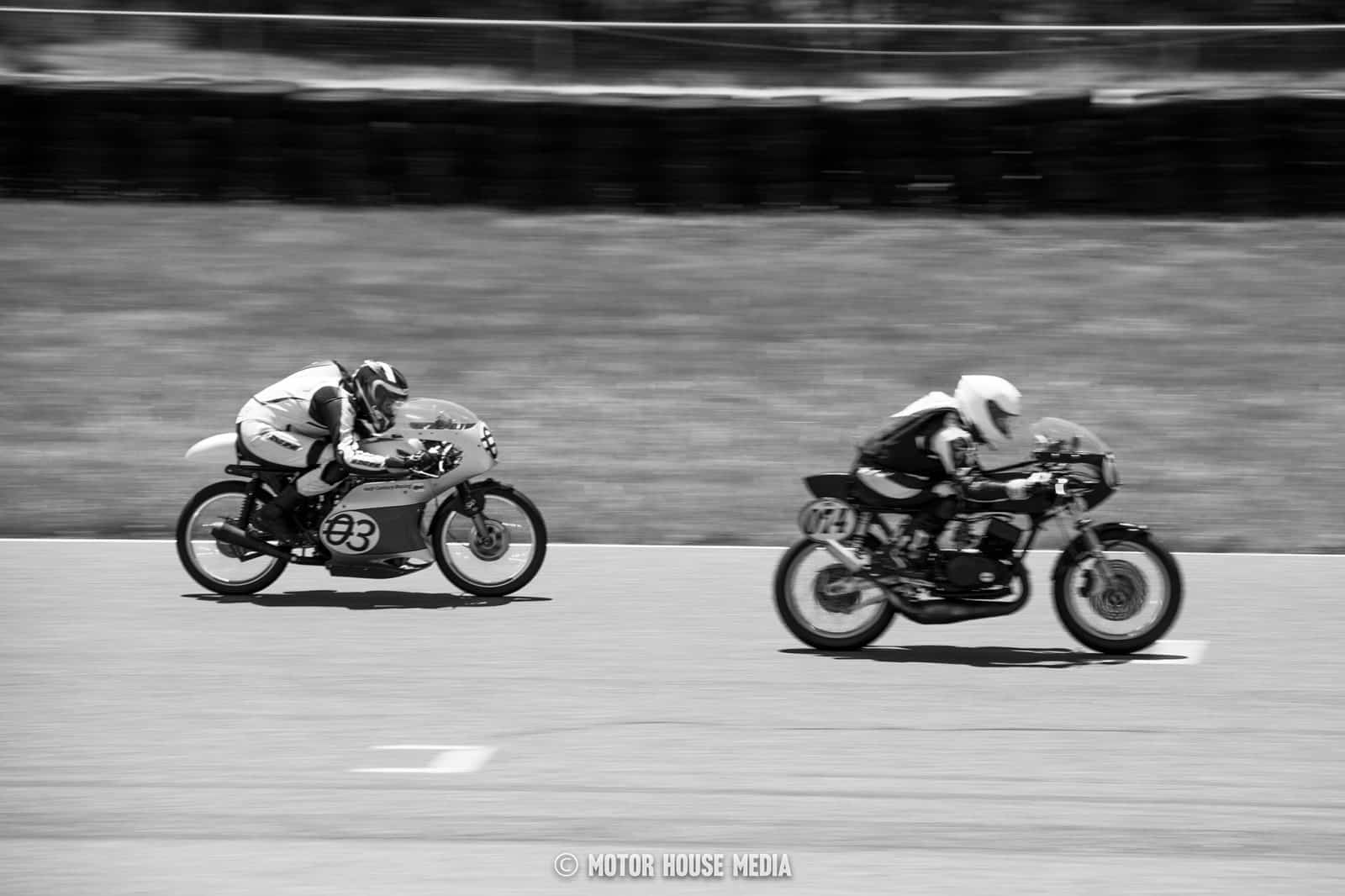This horizontal rectangular black-and-white photograph captures an intense moment during a motorcycle race, showcasing two vintage-style motorcycles that appear to date from the late 1960s or early 1970s. The motorcycles are in sharp focus, while the background blurs into indistinction, emphasizing the high-speed motion of the race. 

In the foreground, the lead motorcycle, bearing the number 074, is ridden by a racer wearing a dark jacket and a white helmet. This rider is crouched low over the black bike to reduce wind resistance. Close behind, the second bike, marked with the number 03, is primarily white, and its rider, dressed in a white jacket and black helmet, is similarly hunched over his handlebars. Their heads are positioned beneath the windshields to maximize aerodynamic efficiency.

The track itself lacks discernible lines, showing only a few white marks here and there. The infield, adjacent to the racing path, is an ambiguous surface—potentially grass—owing to the muted tones of the black-and-white image. Beyond this area, a wall stretches across the scene, with another wall visible at the top of the photograph, suggesting the boundaries of an oval track. The contrasting attire and motorcycles add a layer of visual intrigue, highlighting both the riders' uniformity in technique and their individuality in style.